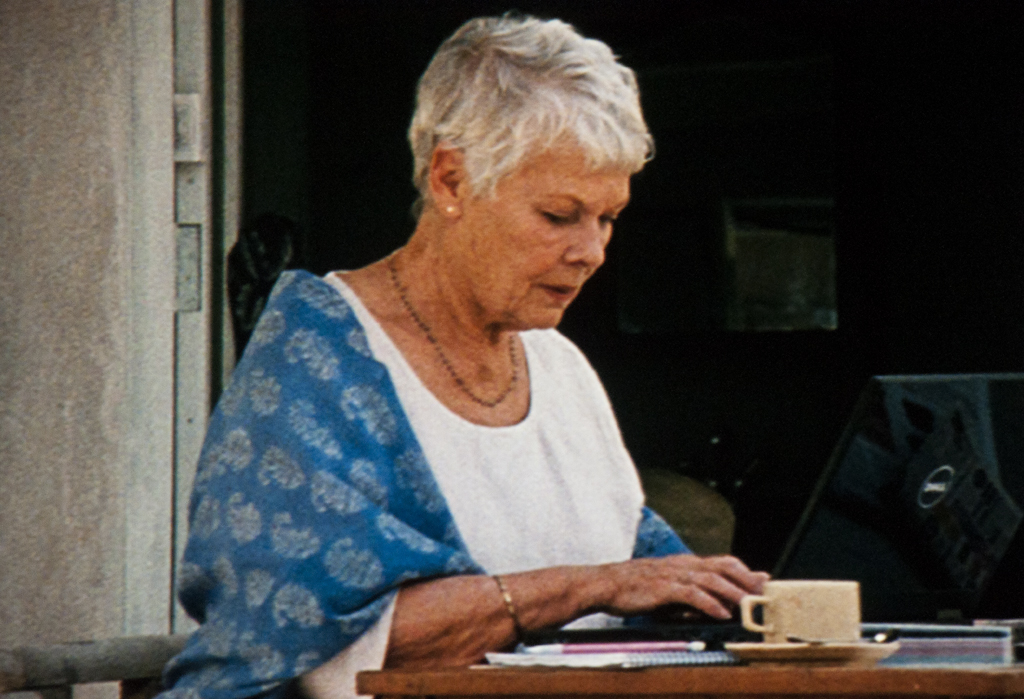The photograph showcases an older woman, likely in her early 70s, sitting at a light brown table. She is the central focus, visible from her lower chest up, and is captured in a grainy, somewhat blurry image. She wears a white short sleeve blouse complemented by a blue shawl adorned with greenish-yellow paisley designs. Her gray hair frames her face, and she accessorizes with a necklace and bracelet. The woman is engrossed in typing on a thin black Dell laptop, with the Dell logo clearly displayed in white on the back.

To the right of her laptop sits a peach-colored small teacup and saucer, with a spoon resting on the saucer. A black bound notebook with a pink and white mechanical pencil lies beside the cup. The overall background is split between a dark, indiscernible space and a whitish-gray door or wall area, adding an element of mystery to the setting. The photo, in its horizontal rectangular format, captures a serene moment of focused activity.